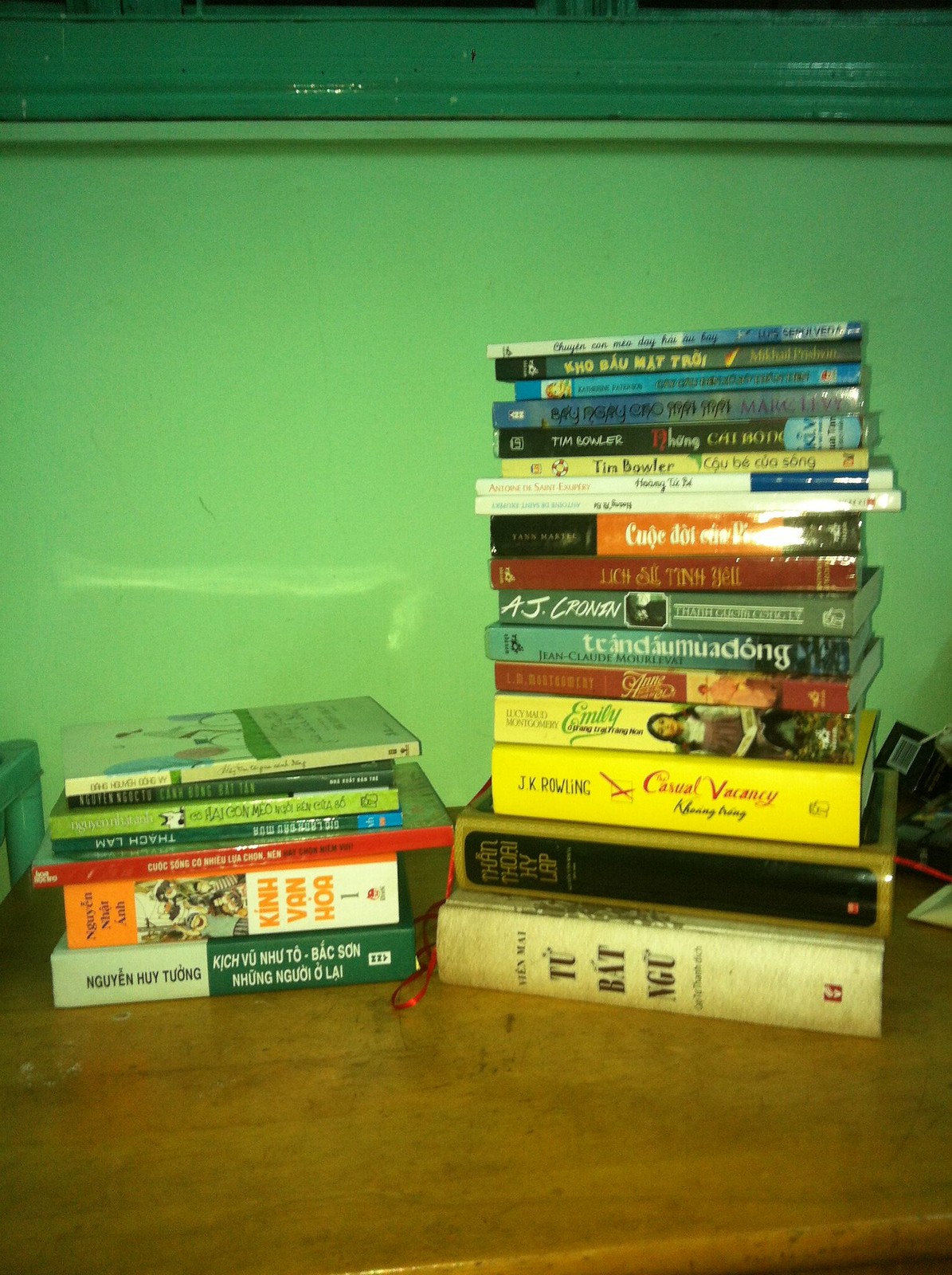The photograph showcases a close-up of a heavily varnished and lacquered wooden desk, revealing its prominent grain and varying shades from oak to darker greys and blacks toward the left. The desk features two distinct stacks of books positioned towards the back; the right stack is significantly taller, about triple the height of the left stack, which contains approximately six books. The spines of these books, some in foreign languages possibly including Vietnamese, are oriented both vertically and horizontally, making it challenging to read all the titles; however, one discernible title is J.K. Rowling's "The Casual Vacancy." The taller right stack begins with a thick white hardbound book at the bottom, followed by another thick book and several paperbacks of varying thicknesses stacked on top. The backdrop of the image includes a green painted wall with noticeable scuffs and, possibly, a deeper green-colored wooden window ledge or a metallic-like structure.